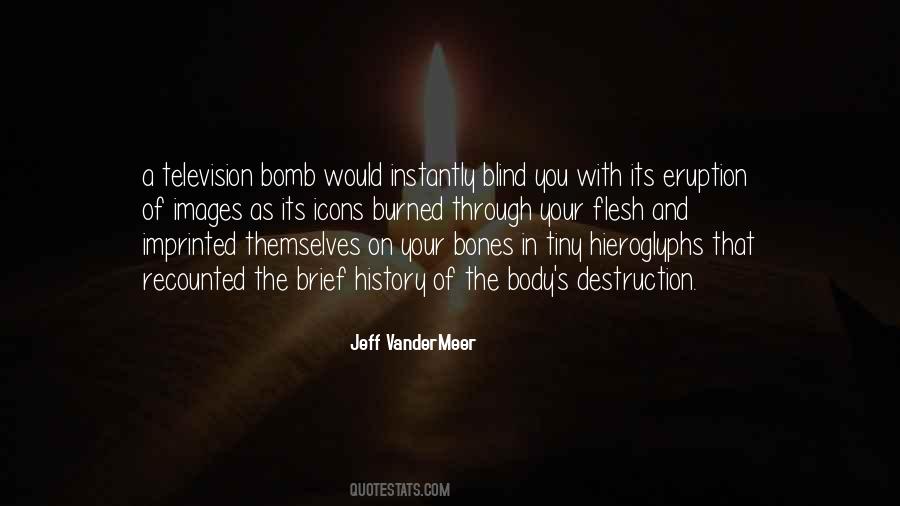The image features a dark background with a faint, dimly lit scene of an open book and a small candle, the candlelight softly illuminating the pages. Superimposed over this backdrop is a striking, bright white handwritten text that reads: "A television bomb would instantly blind you with its eruption of images as its icons burned through your flesh and imprinted themselves on your bones in tiny hieroglyphs that recounted the brief history of the body's destruction." Below this evocative quote is the name "Jeff VanderMeer," followed by "QUOTESTATS.COM" in uppercase. The scene creates a haunting contrast, emphasizing the surreal and destructive nature of the written words.